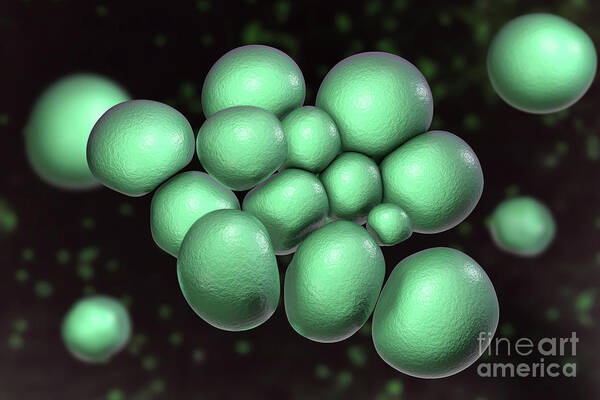The digital art piece showcases a collection of bright, almost neon green, spherical shapes, reminiscent of molecules or grapes, grouped together in the center of a black background. These orbs vary in size and form, with some being perfectly round while others appear slightly oblong. The cluster is visually striking, evoking a sense of otherworldly or microscopic life forms due to their seemingly poisonous hue. Around the main cluster, a few smaller orbs are scattered, providing a sense of depth and space within the image. Notable among these is a larger green orb in the top right corner. In the lower right-hand corner, a transparent white watermark reads, "Fine Art America," adding a subtle signature to the piece. The background fades into darkness, with additional green shapes disappearing into the void, suggesting an expansive, unseen field of these vivid forms.